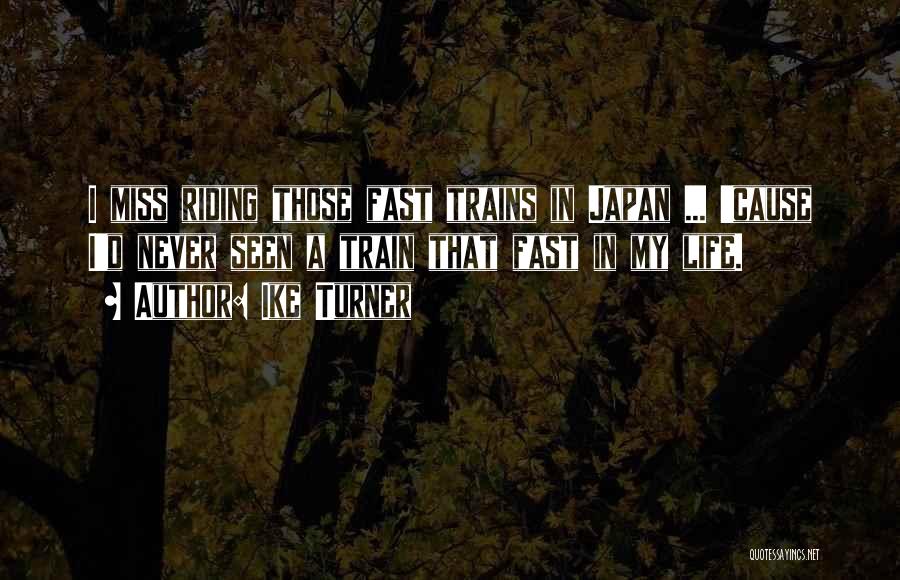The image is a very dark, almost blackened photograph, as if a filter or film has been applied. It features a forest full of fall-like trees with visible trunks and branches adorned with yellow and some orange leaves. Superimposed over the image are black block letters with white borders, and each word is enclosed in a white rectangular space. The text reads, "I miss riding those fast trains in Japan, because I'd never seen a train that fast in my life, Arthur Ike Turner." In the bottom right corner, there is a tag in white letters that reads "quotes sayings dot net."